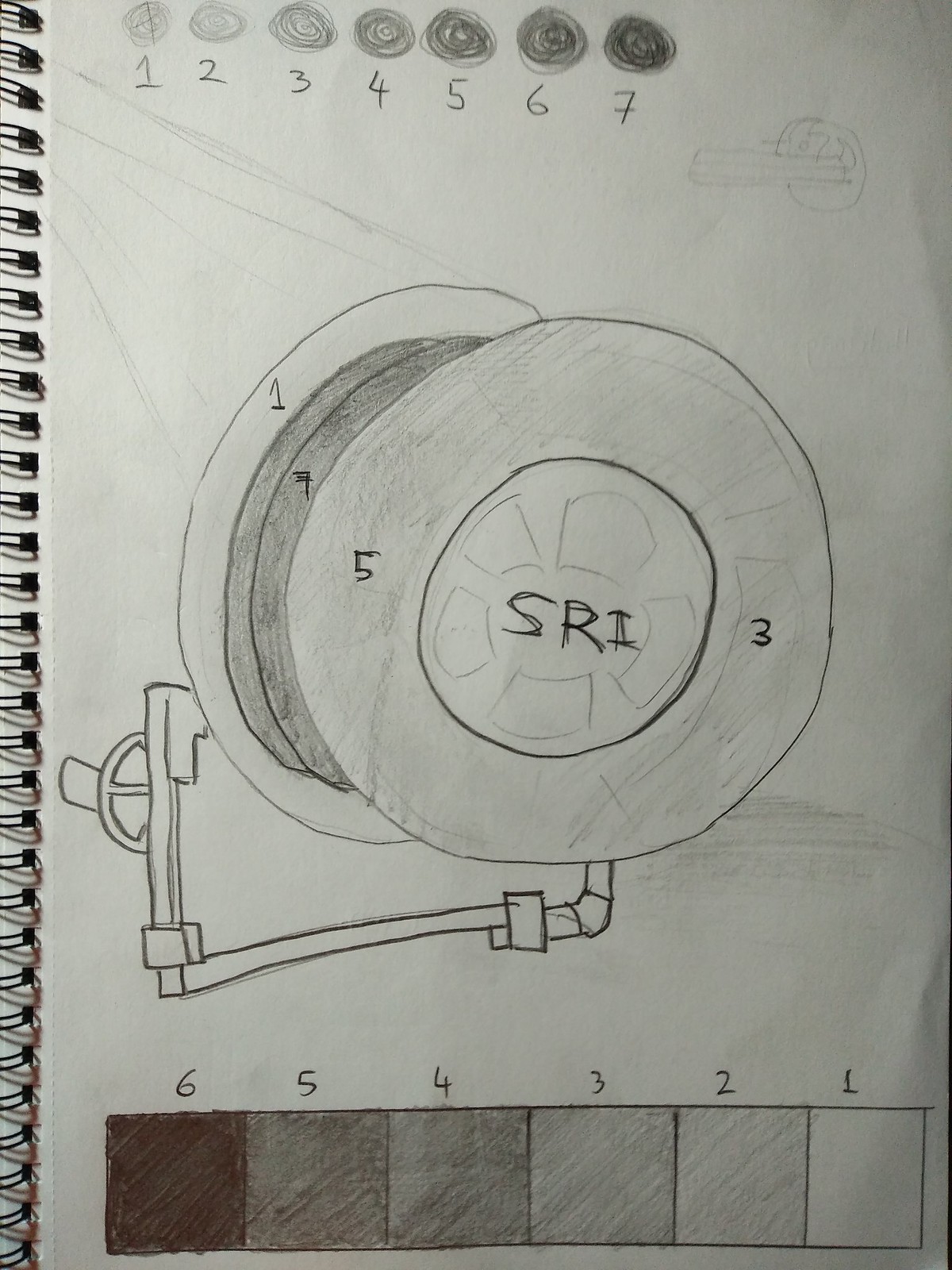The drawing appears to be a detailed hand-drawn illustration created using pencil on a white sheet of paper. At the top of the image, there are seven circles aligned horizontally. Each circle is labeled with numbers from one to seven, starting from the left. The circle above number one is the lightest in shade, and each subsequent circle progressively darkens, with the darkest circle above number seven.

Below these circles, the primary focus of the image is a large spool, similar to those used to wind garden hoses. Written across the spool are the letters "SRI". A garden hose seems to be wrapped around this spool, suggesting its purpose in the illustration.

Further down, there is a depiction of a pipe or conduit extending below the spool. Attached to this pipe is a round handle, indicating that it can be turned, likely to control the flow of water through the pipe.

At the very bottom of the image, there are six squares arranged in a row, each marked with a number from one to six. The square marked with number six is the darkest, and the shading of each consecutive square lightens incrementally until the square marked with number one, which is the lightest of all.

This meticulous drawing uses shading and labeling to convey a detailed and intricate mechanical object, possibly emphasizing the gradation in shading and the functionality of the components depicted.